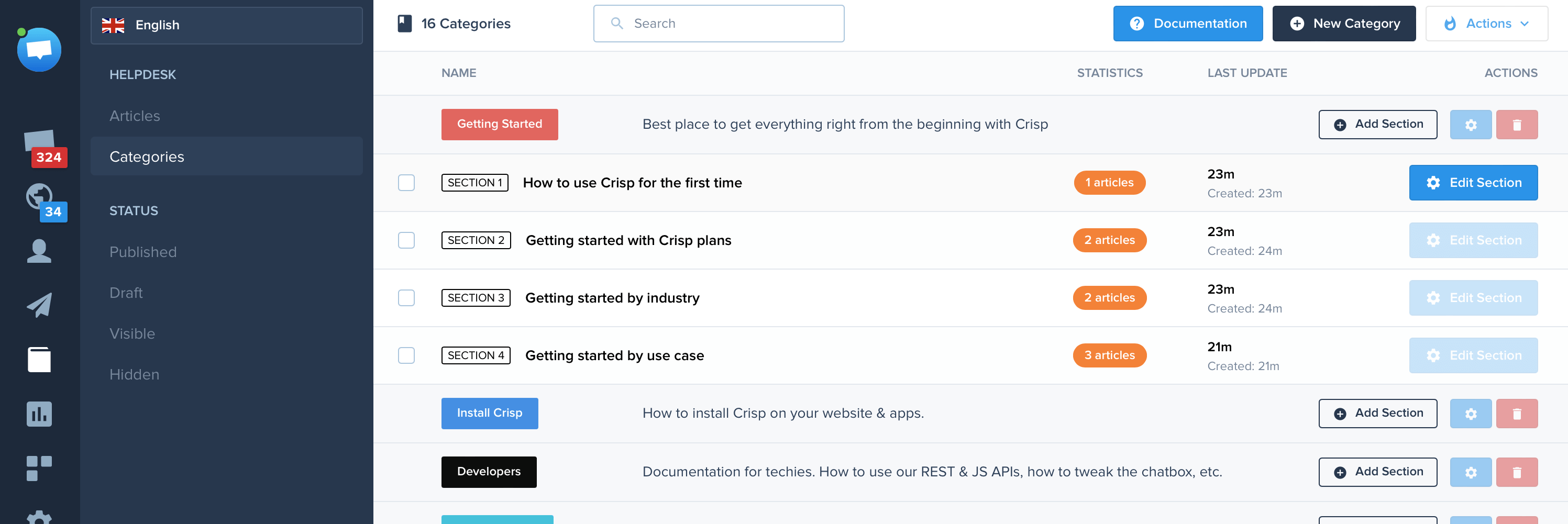The image depicts a screen with a user interface for managing categories in a content management system. On the far left is a vertical grey panel containing a series of icons at the top, followed by an English flag icon and the word "English." Below these are various menu headings including "Helpdesk," "Articles," "Categories," "Status," "Published," "Draft," "Visible," and "Hidden," with the "Categories" option currently selected.

Occupying the majority of the screen to the right, the main category management area is shown. At the top of this section is a white banner displaying a counter that indicates "16 categories." Next to this is a search bar for entering search criteria. Adjacent to the search bar are a blue "Documentation" button, a grey "New Category" button, and a white "Actions" dropdown menu.

Below the banner is a grid with columns labeled "Name," "Statistics," "Last Update," and "Actions." Under the "Name" column, several categories are listed such as "Getting Started" (highlighted with a red button labeled "Getting Started"), and "Section 1" through "Section 4," each accompanied by checkboxes that can be selected. The "Statistics" column shows the number of articles associated with each category. For instance, the "Getting Started" category is linked to one article, indicated by a small orange button on the right-hand side.